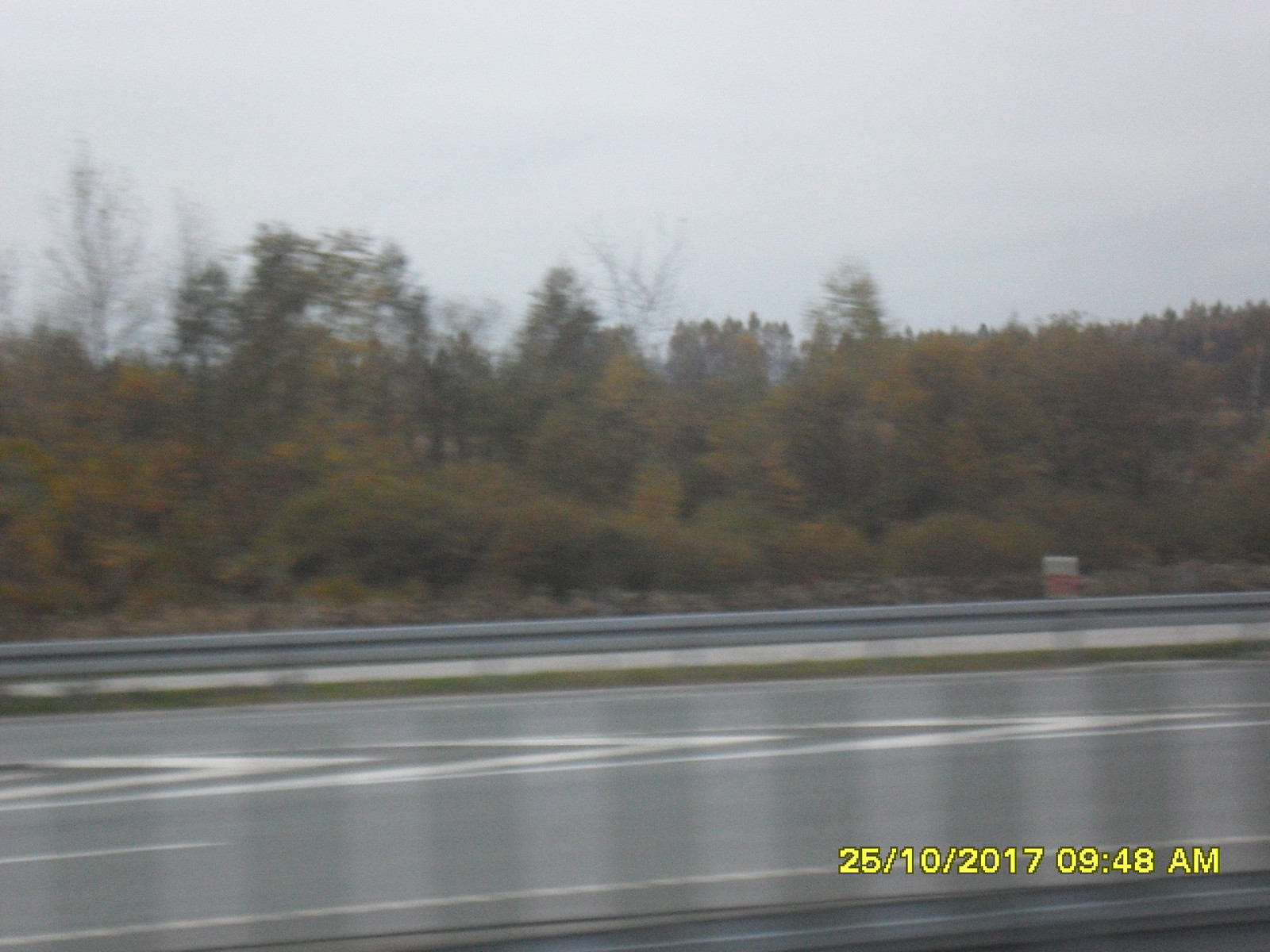This photograph captures a moment on a two to three-lane road, possibly mistaken for a highway, taken from the side of the street. The timestamp "25-10-2017 at 09:48 a.m." is prominently displayed in yellow in the bottom-right corner. The foreground shows some pavement with faint white markings, indicating road lines. On the opposite side, a gray barrier runs along the edge of the road, separating it from a row of brownish-green trees, which add a touch of nature to the scene. The sky is overcast, suggesting a gloomy or rainy day. Additionally, there is a small box-like structure in the distance on the other side of the road, colored in orange and white, its purpose unclear from the image.